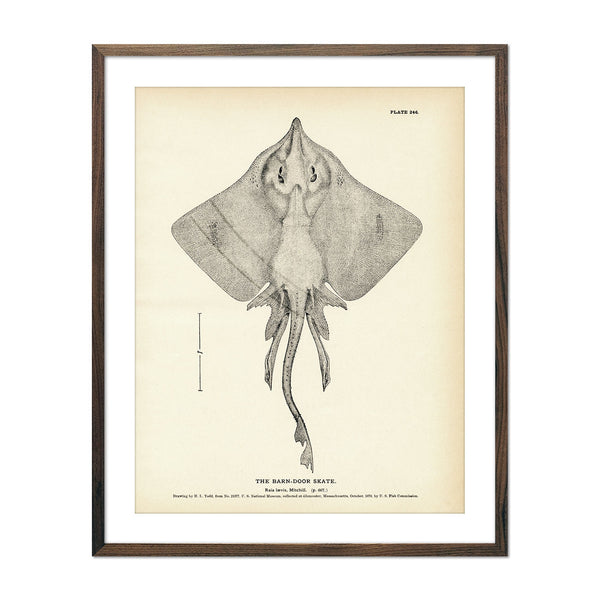This framed artwork features a detailed, black-and-white technical drawing of the underside of a barn door skate, a marine creature similar to a stingray. The animal's diamond-shaped body is prominently displayed, with its wings extending outwards and an elongated tail featuring various segments. At the top of the drawing are the eyes, and towards the bottom, the tail stretches out, nearly matching the body in length. The illustration appears to be from a scientific book or textbook, set against parchment or slightly discolored paper. Below the image, there is text labeling the creature as the "barn door skate," along with additional annotations such as "plate something" and a scale number. The precise and intricate depiction of the skate showcases the significant anatomical details, making it both an educational piece and a work of art.